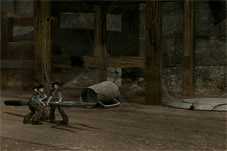This intricate and richly detailed artwork, possibly a painting or a graphic from a video game, features a small, rectangular, predominantly brown image. In the foreground, three diminutive figures dressed in brown pants appear to be cowboys or young men. They are collectively holding a massive, rudimentary-looking cup with a handle, angled like a large brown mug. The object they are holding is described variously as a tool, a knife, or a beam, but its shape is most clearly discerned from its shadow on the dark brown wooden floor — a pitchfork or large fork.

In the background, the scene incorporates a mix of furniture or structural elements, including vertical and horizontal brown pieces that resemble part of a chair or wooden framework, alongside a grayish-brown brick wall. The composition hints at a large, wood-themed building or cupboard, contributing to the diminutive appearance of the figures compared to their surroundings and the enormous cup they are handling.